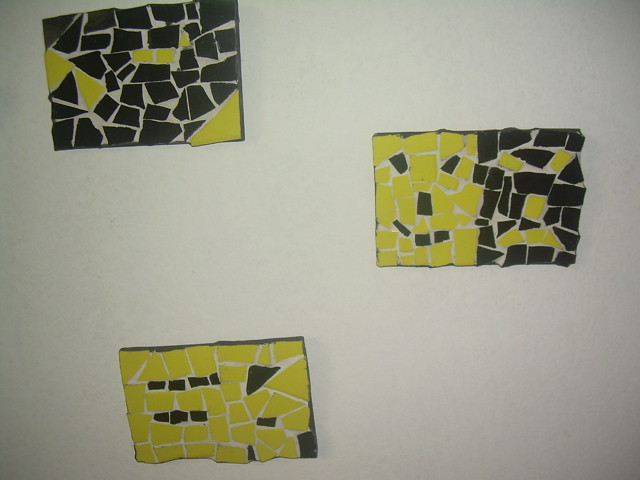The image features a wide rectangular artwork installation on an off-white wall, which fades to a grayish tone towards the lower corners. The installation includes three distinct pieces. The top left piece is a rectangular artwork slightly angled upward, composed mainly of dark green tiles arranged in a mosaic pattern, with a few yellow tiles interspersed. Below this, towards the bottom center but slightly to the right, is another rectangular collage dominated by light yellowish-green tiles, with just a few dark green ones scattered throughout, giving it a flag-like appearance. The third piece is centrally positioned to the right and features a split design with a smiley face on the left side with a yellow background and a grumpy face on the right side with a dark green background, both bordered by white outlines. All three pieces, made up of various shapes and sizes of tiles, create a visually intriguing, minimalist mosaic artwork display.